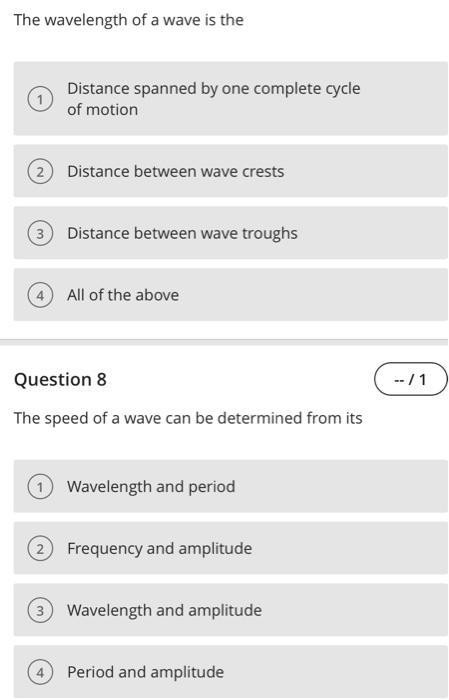The image is a digital screenshot showcasing a question-and-answer interface, likely from either a mobile app or a website. At the top of the screen, it displays the question, "The wavelength of a wave is the:" followed by four possible answers: 

1. Distance spanned by one complete cycle of motion.
2. Distance between wave crests.
3. Distance between wave troughs.
4. All of the above.

Each answer is enclosed within its own gray rectangle and marked with a gray circle containing the answer number to its left.

Below this question is another one, labeled as question eight. To its right, a circular icon indicates a dot and displays "0/1," signifying that no questions have been answered out of one possible question. The eighth question posed is, "The speed of a wave can be determined from its:" with the following options:

1. Wavelength and period.
2. Frequency and amplitude.
3. Wavelength and amplitude.
4. Period and amplitude.

Similar to the previous question, each answer is contained within a separate gray rectangle and numbered within a gray circle. The overall background of the web page is stark white, providing a clean and uncluttered look.